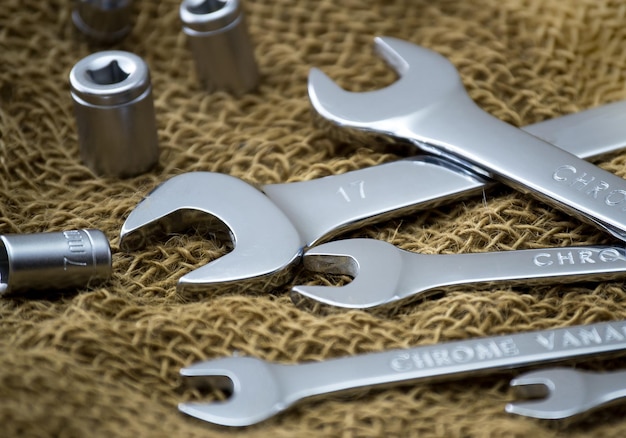The image displays a variety of silver tools arranged on a brown net material. Prominently featured are five wrenches of different sizes, including a 17mm wrench and a larger one, with the smallest on the side. Inscribed on the wrenches is the word "chrome." Additionally, there are four nuts on the left side, one of which is marked as 7mm. The scene also includes sockets, highlighting their utility in fitting screws in hard-to-reach areas. This collection of tools underscores their indispensable convenience and utility.